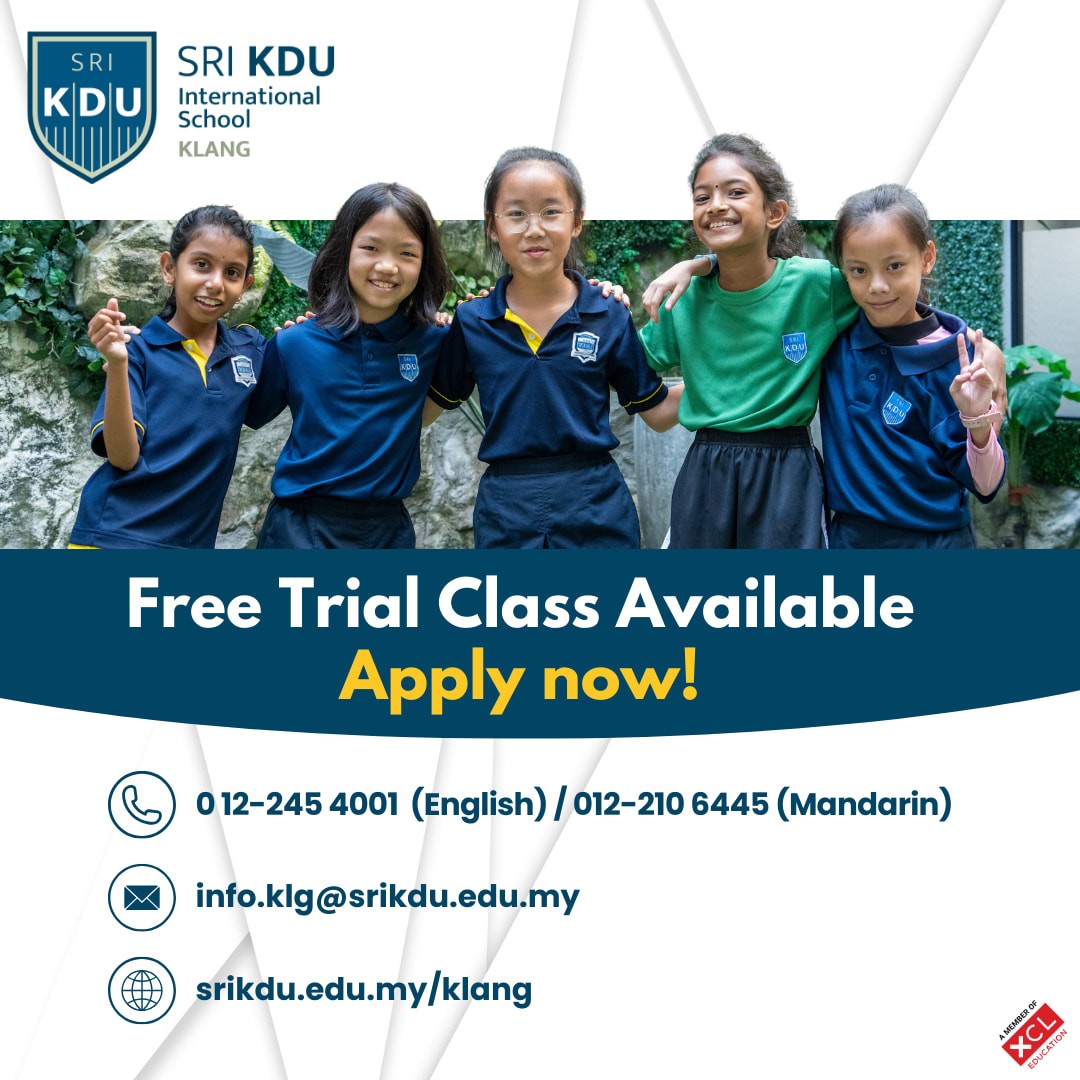The image features a white background with an icon resembling a shield in the top left corner. The shield displays the text "SRI KDU" with vertical lines between the letters. To the right and slightly below the shield, the words "SRI KDU International School Klang" are prominently written. 

Beneath this text are five girls wearing school outfits that resemble soccer uniforms, illustrating the school's active student participation. Below the image of the girls, a promotional message reads "Free trial class available now. Apply now."

In the lower section, contact information is provided with various icons for clarity. A telephone icon is followed by: 
- "012-245-4001" with "English" in parentheses.
- "012-210-6445" with "Mandarin" in parentheses. 

Additionally, an envelope icon precedes the email address "info.klg@srikdu.edu.my." Lastly, a globe icon indicates the school’s website: "srikdu.edu.my/klang."